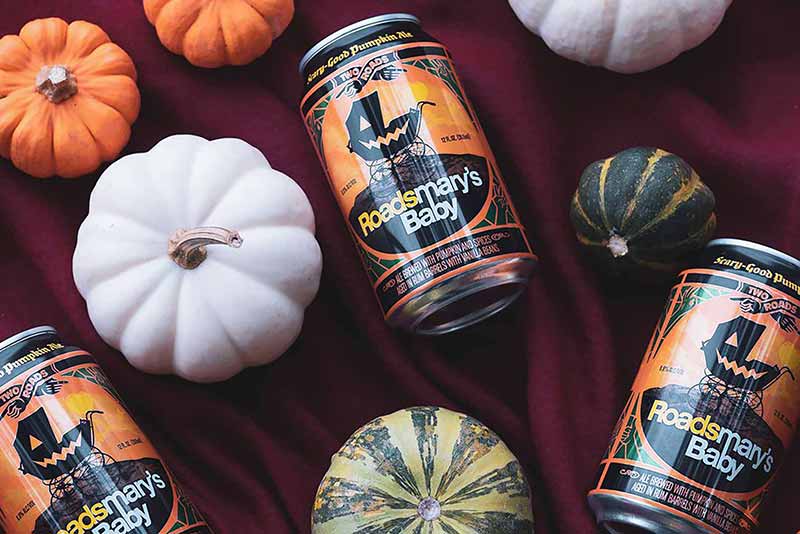This overhead photograph features an advertisement setup for Rhodes Mary's Baby's Scary Good Pumpkin Ale, a product of Two Roads Brewery. The scene is set on a wine-colored velvet cloth, with three cans of the ale lying on their sides, each showcasing a black, old-time baby carriage with jack-o'-lantern facial features on the front. The text on the cans reads "Rhodes Mary's Baby" in orange and black graphics, with additional descriptors including "brewed with pumpkin and spices aged in rum barrels with vanilla beans."

Around the cans, a variety of pumpkins are artistically arranged. The top section of the image features two small orange pumpkins to the left and a white pumpkin below them. The bottom center showcases a green melon-like pumpkin, while the right section has another white pumpkin and a green-yellow pumpkin below it. The pumpkins and squash create a festive and visually appealing Halloween-themed display, enhancing the overall autumnal, spooky ambiance of the advertisement.